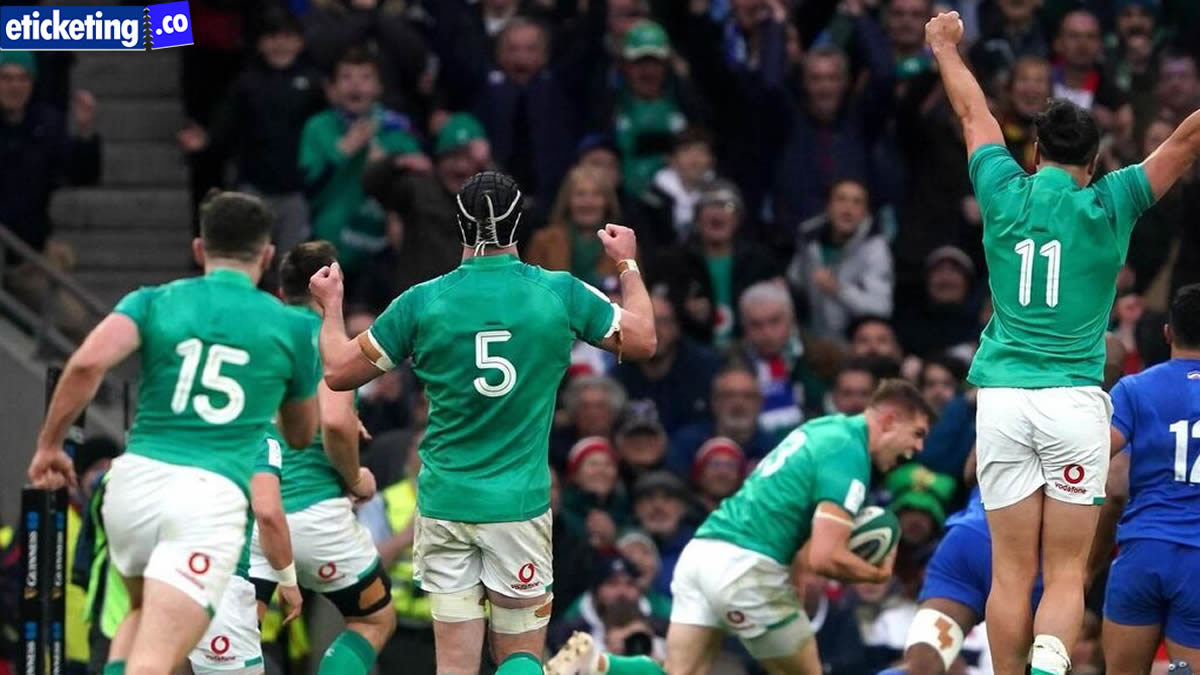The image depicts a vibrant and thrilling moment during a rugby match between two teams—the green team and the blue team—captured in a large stadium filled with cheering spectators. The green team, wearing green short-sleeved tops and white shorts branded with the Vodafone logo, dominate the scene. Central to the image is player number 15 from the green team, running with his back to the viewer, as he advances towards the opposing team's territory. To the left, player number 5 from the same team has his hands raised, possibly in celebration of a recent score. In the foreground, a green team player, mouth open in a determined shout, grips the rugby ball tightly as he charges forward, while player number 11 on his team raises his arms in triumph. Meanwhile, on the right side of the image, two players from the blue team, dressed in blue shirts and shorts, including number 12, brace themselves for the impending tackle. The excitement of the crowd in the blurred background, coupled with the eTicketing.co banner visible on the left-hand side, underscores the electric atmosphere of this high-stakes sporting event.